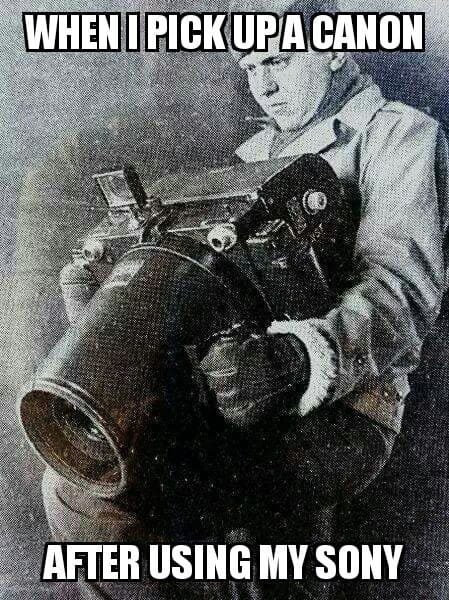The image is a black-and-white advertisement with a grainy texture, reminiscent of an old photograph from the 1940s. At the center of the image stands a man dressed in a military-style hat, scarf, light jacket, and dark pants, complemented by thick winter gloves. He holds an enormous camera with a black body, a viewfinder extending from the top, and a very long lens that he supports with his left leg. The camera is so large that it stretches from his chest to beyond the reach of his arms. Superimposed text in a white block font reads "When I pick up a Canon" at the top, and "after using my Sony" at the bottom, playing humorously on the perceived heaviness of Canon cameras compared to Sony. The positioning of the text at the top and bottom frames the central image in a style similar to a meme or postcard, reinforcing the comedic tone.